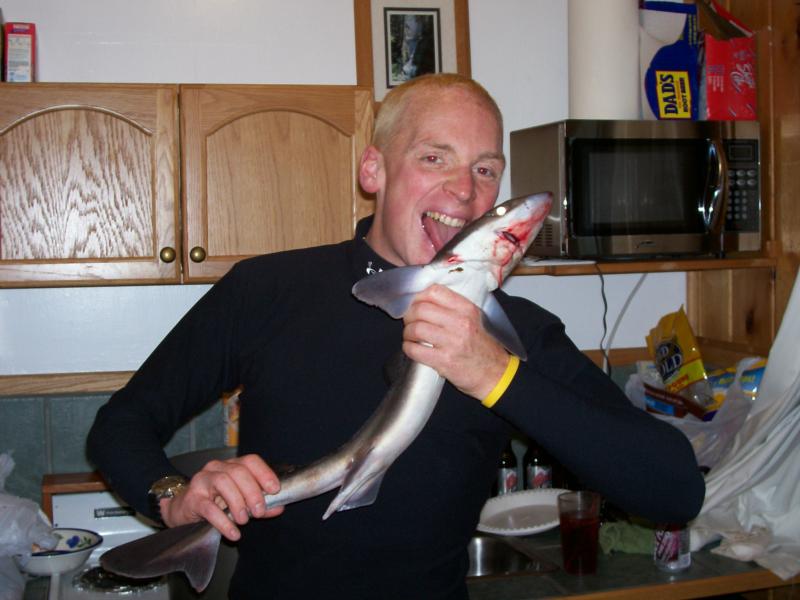In this indoor photograph, a cluttered kitchen serves as the backdrop. Central to the image is a man with very short blonde hair and red pupils, who is wearing a black long sleeve Under Armour t-shirt. On his right wrist, he sports a gold watch with a black band and on his left wrist, a yellow Livestrong rubber bracelet. The man, who occupies the center of the image, is holding a small, bloody shark with a white belly and silver-gray skin. He is playfully licking the shark's head while looking directly at the camera. 

The background reveals light brown wooden cabinets and a congested blue-gray counter littered with beer bottles, a silver and red soda can, a white plastic plate, a glass of red juice, grocery bags, garbage, and bags of chips. A wall adorned with green splash tiles can also be seen. To the right, a silver microwave sits on a wooden shelf, topped with a roll of paper towels and boxes of Dad's Root Beer and Shasta Cola. A white stove is partially visible along with a box on top of one of the cabinets on the upper left. There’s also a picture hanging on the wall in the center. The predominant colors in the image are white, red, blue, black, yellow, orange, and gray, contributing to the overall chaotic yet vibrant scene.